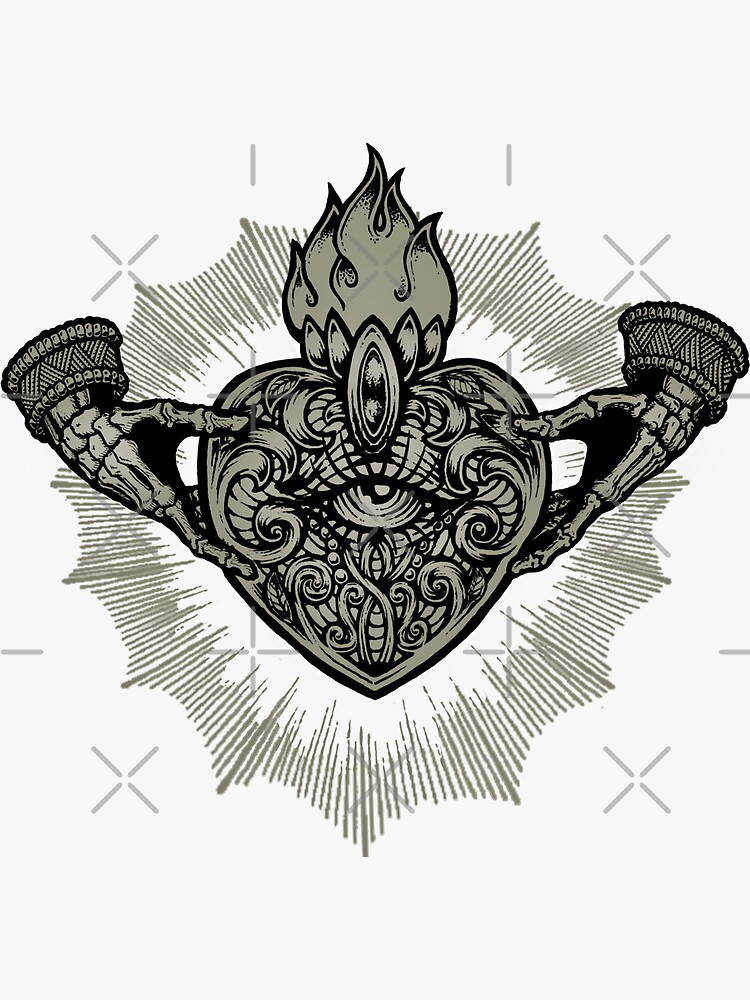This intricate black and brown line drawing, reminiscent of an emblem or badge and possibly intended as a tattoo design, is set against a white background with a subtle grayish tint. At the center, it features a heart with an open human eye adorned with detailed eyelashes and various swirled patterns. Mounted above, the heart appears to wear a flaming crown, with flames intricately rising from the top. Flanking the heart on both sides are two skeletal hands, each wearing elaborate cuff sleeves that resemble intricate beadwork, consisting of two rows of beads encircling a central beaded section. Surrounding the entire composition are a series of X's and additional line patterns, adding an ornamental border to this already detailed piece.